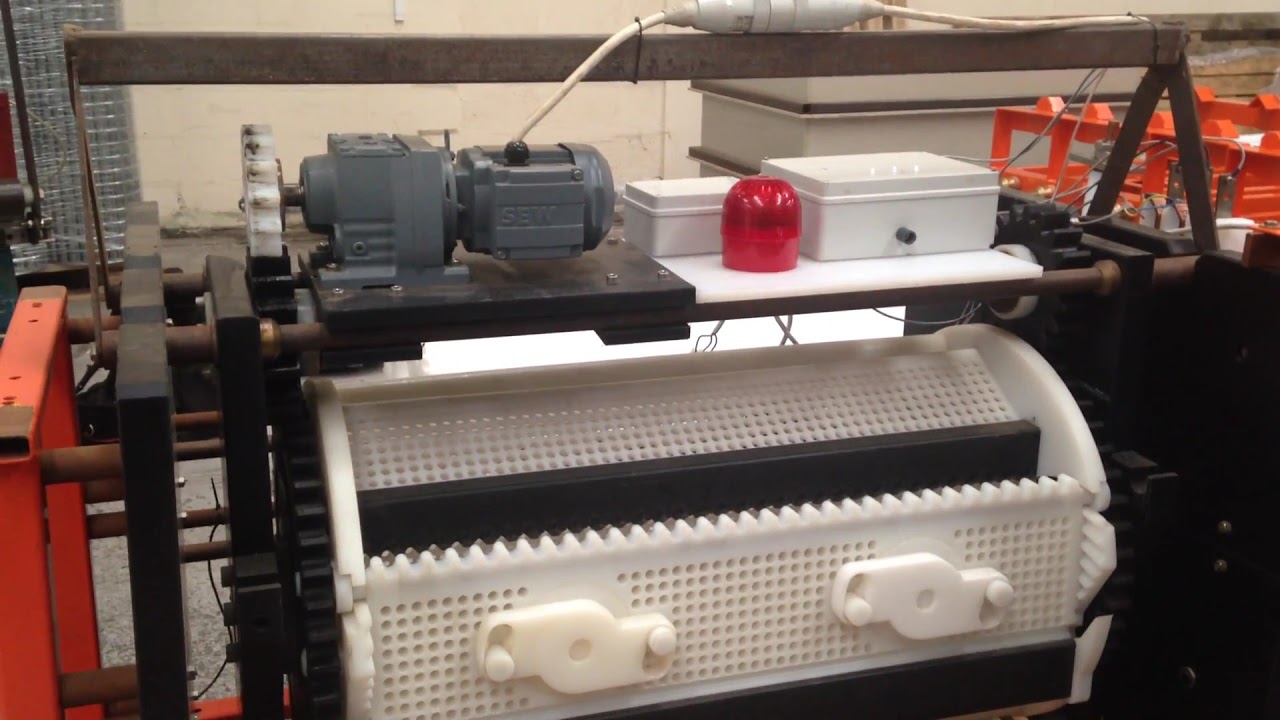The image showcases a complex machinery setup that appears to belong to a workshop, maker's studio, or science lab. At the bottom, there's a large white component resembling a scaled-up version of a toy car engine. This part has a smooth, plastic-like exterior dotted with numerous tiny holes on one side. Projecting from it are two buttons, which secure a plastic piece in place. The machinery is framed by a more robust, metallic structure, giving an impression of industrial-grade equipment.

Within this structure, there's another smaller engine featuring white gears interlocked with darker gears, which connect to the larger engine described earlier. 

Above this setup, a black table or desk supports several items: two white metal boxes of different sizes, a red cylindrical or spherical object, and a grey device that looks like a motor. The grey item is branded with "SBW" and is tethered by a thick wire. To the right, within an orange frame, some additional parts of the machinery are visible, while a detail along the top right shows a porridge crate.

This intricate array of machinery, accessories, and additional components gives a sense of a sophisticated and functional workspace, possibly involved in precision engineering or scientific experiments.